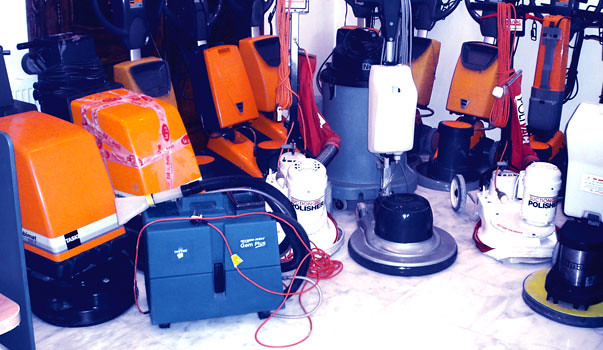In this slightly faded and overexposed landscape-oriented photograph, we see a collection of various floor buffing and polishing machines, arranged closely together and occupying most of the frame. The image quality isn't the best, with noticeable overexposure, especially a large white hotspot near the foreground center, obscuring details. The devices are set against a backdrop of white marble flooring with grey striations, and a plain white wall. 

Among the machines, a few distinct types are identifiable: one has a silver circumference around its base, a black motor head, and a white tank along its vertical rod for holding it. Most units, however, are orange with black caps, indicating they are used for some form of cleaning or polishing. Additionally, there is an orange piece with tape on it, suggesting it might be broken. A smaller white polisher plainly marked "polish" stands out among these machines. 

Electrical cords, predominantly red and orange, are coiled up and hang down onto the floor, adding to the cluttered atmosphere. One particular machine near the front features a yellow disc and a black cleaning mechanism, possibly a different type of floor cleaning equipment. The faded photograph, apparently from the 60s or 70s, captures 13 machines in total, with their backs to the wall but facing towards the camera, hinting at a storage area for these cleaning devices.